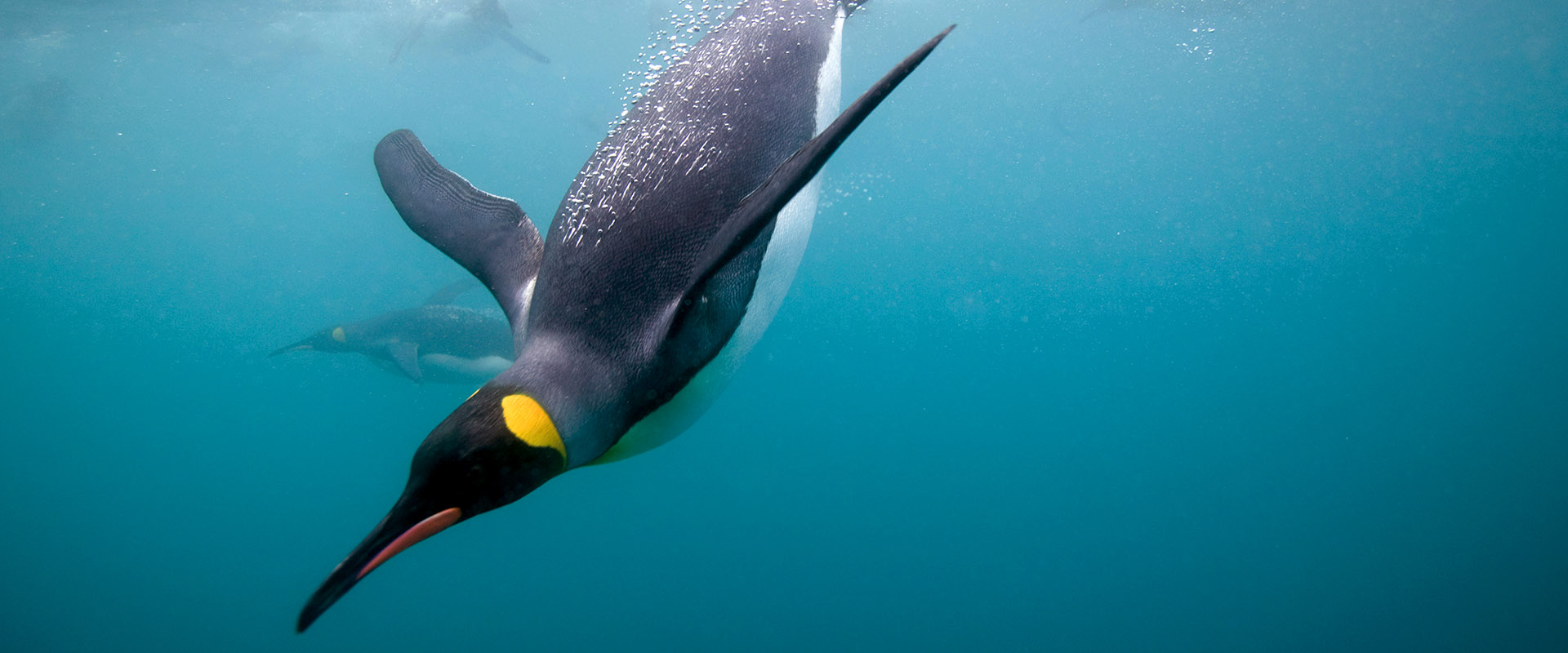An underwater photograph captures the striking scene of a penguin diving into the murky, dark blue ocean, with bubbles trailing off its back, indicating it has just freshly plunged in. The penguin, which is the primary focus of the image, is situated slightly to the left of the center. It boasts a black back, a white belly, a yellow spot on its neck, and a sharp, elongated bill with some red or peach accents noticeable on the underside. The wings of the penguin are extended wide as it heads downward. Behind the main penguin and further in the background, at least one more penguin is visible swimming, slightly blurry due to the distance. The far top right of the image shows an indistinct shape, potentially another swimmer, whether human or penguin, leaving a notable trail of bubbles. The photograph’s composition and the details of the penguin such as its black and white coloration and splashes of yellow make it likely to be an Emperor penguin, although its precise species is not clearly determinable from the image alone. The water surrounding the penguins appears deep and peaceful, adding to the photograph's tranquil yet lively atmosphere.